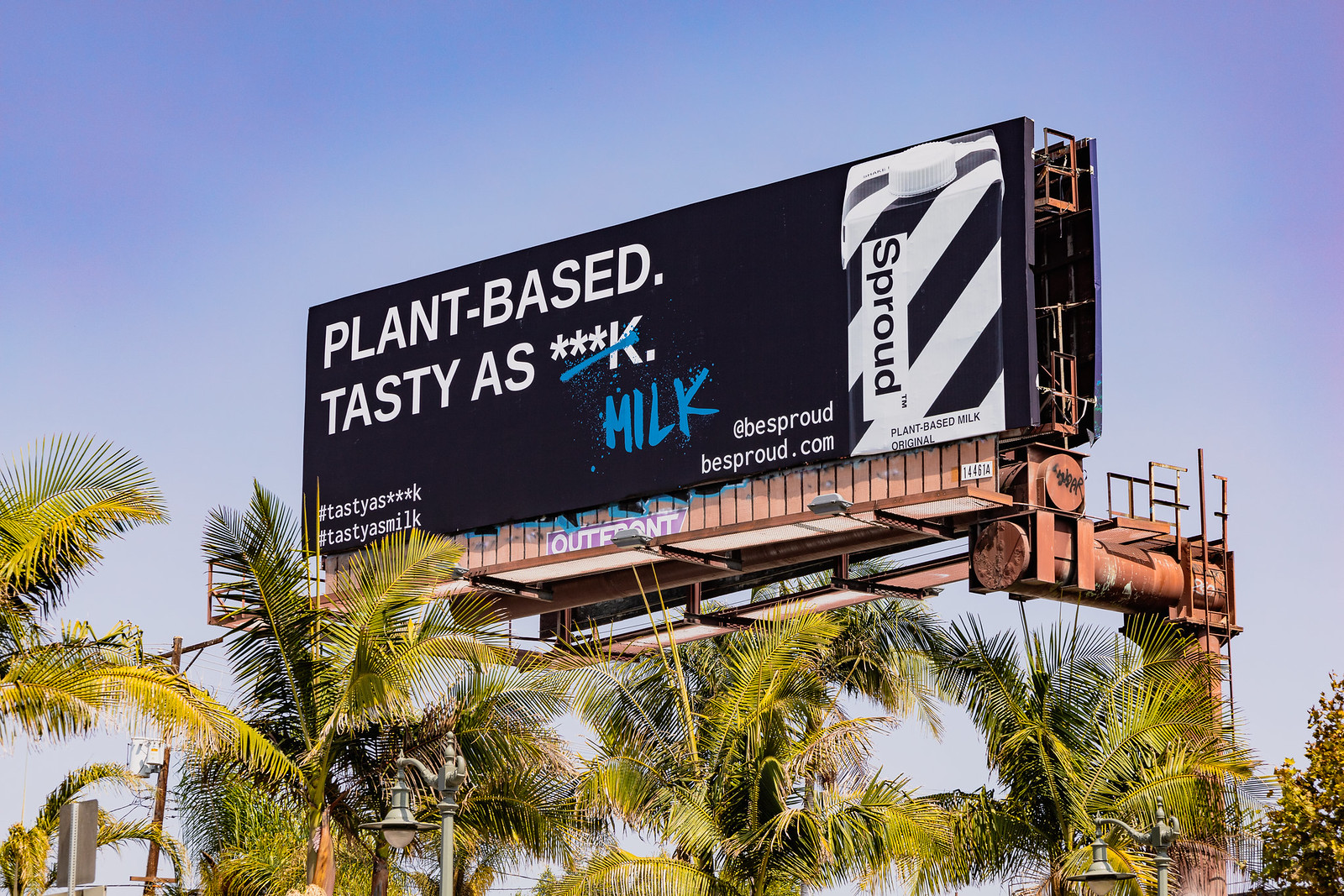This image showcases a dynamic, upward-angled view of a billboard elevated high above a grove of palm trees. The billboard is mounted on a robust red metal structure, with a prominent round red pole serving as its main vertical support. Attached to the pole is a ladder that ascends to the top of the billboard.

The billboard itself features a bold design with a black background. In the top left corner, white text reads "Plant-based, tasty as ***k," with a blue, graffiti-style spray-painted line crossing through it. Below this modified slogan is the word "milk," appearing as if it were also spray-painted.

In the bottom left corner, the billboard displays two hashtags: "#tasty as ***k" and "#tasty as milk." Dominating the right side is a large image of a black-and-white striped carton of milk. The carton is labeled "Sprout" vertically down its side, and at the bottom, it reads "Plant-based Milk, Original" in black letters.

The entire scene is set against a clear, cloudless blue sky, which serves as a striking backdrop and highlights the vivid colors and details of the billboard.